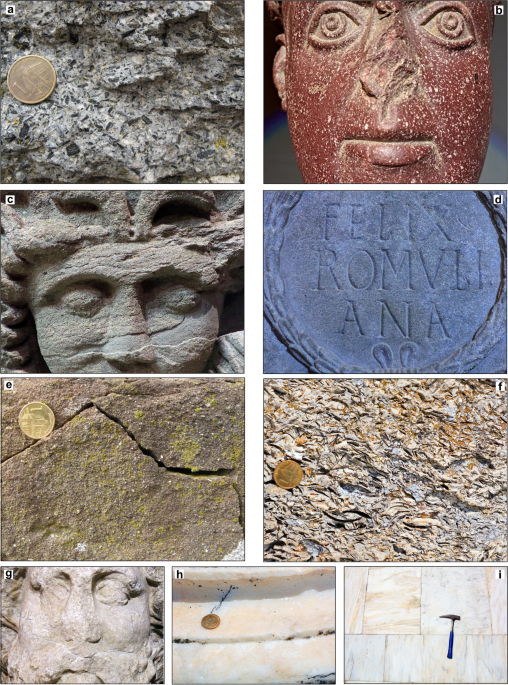This image features a grid of nine labeled color photographs (A through I), each highlighting different ancient stone artifacts with varying states of preservation, typically accompanied by a coin for scale. 

- **A**: A rough, gray stone surface with a small bronze coin placed on it for scale. 
- **B**: A carving of a face in a red stone with white spots, missing its nose.
- **C**: A detailed gray stone face sculpture with rounded eyes and a pointed design around the head, appearing weathered and ancient.
- **D**: A bluish-gray stone with an inscription, "Felix Romula Anna," engraved in a circular pattern and surrounded by a laurel wreath.
- **E**: A brownish stone with a deep black crack and a mossy green tinge, featuring a gold coin in the top left.
- **F**: A mottled gray and brown stone surface with a copper coin in the middle left of the frame.
- **G**: A stone face sculpture showing a beard and curly hair, appearing quite worn and ancient.
- **H**: A brownish-white marble surface with a copper coin in the center left.
- **I**: Light brown and white-mottled marble tiles with a hammer or chisel with a black head and blue handle positioned to the right.

These images collectively display an array of stone artifacts and carvings, primarily faces and inscriptions, with notable diversity in color, texture, and condition, highlighting their ancient and historical significance.